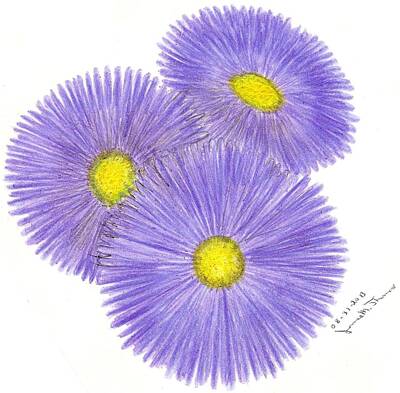The image displays a detailed and realistic painting, likely hand-drawn, of three Asteraceae flowers with fine, purple petals and a rich, egg yolk yellow center. The flowers, which resemble purple dandelions or fleabane, are set against a clean, white background, giving emphasis to their intricate structures. The petals, described as "rays," extend delicately from the flower's core, where the yellow center, housing what appears to be seeds, stands out. The painting's artistic strokes and lifelike depiction suggest a high level of skill. A signature in black is located at the bottom right corner of the image, adding a personal touch from the artist. The overall composition suggests a nature-focused theme, set to capture the pure beauty of these floral elements perhaps as seen from a window or imagined in still life.